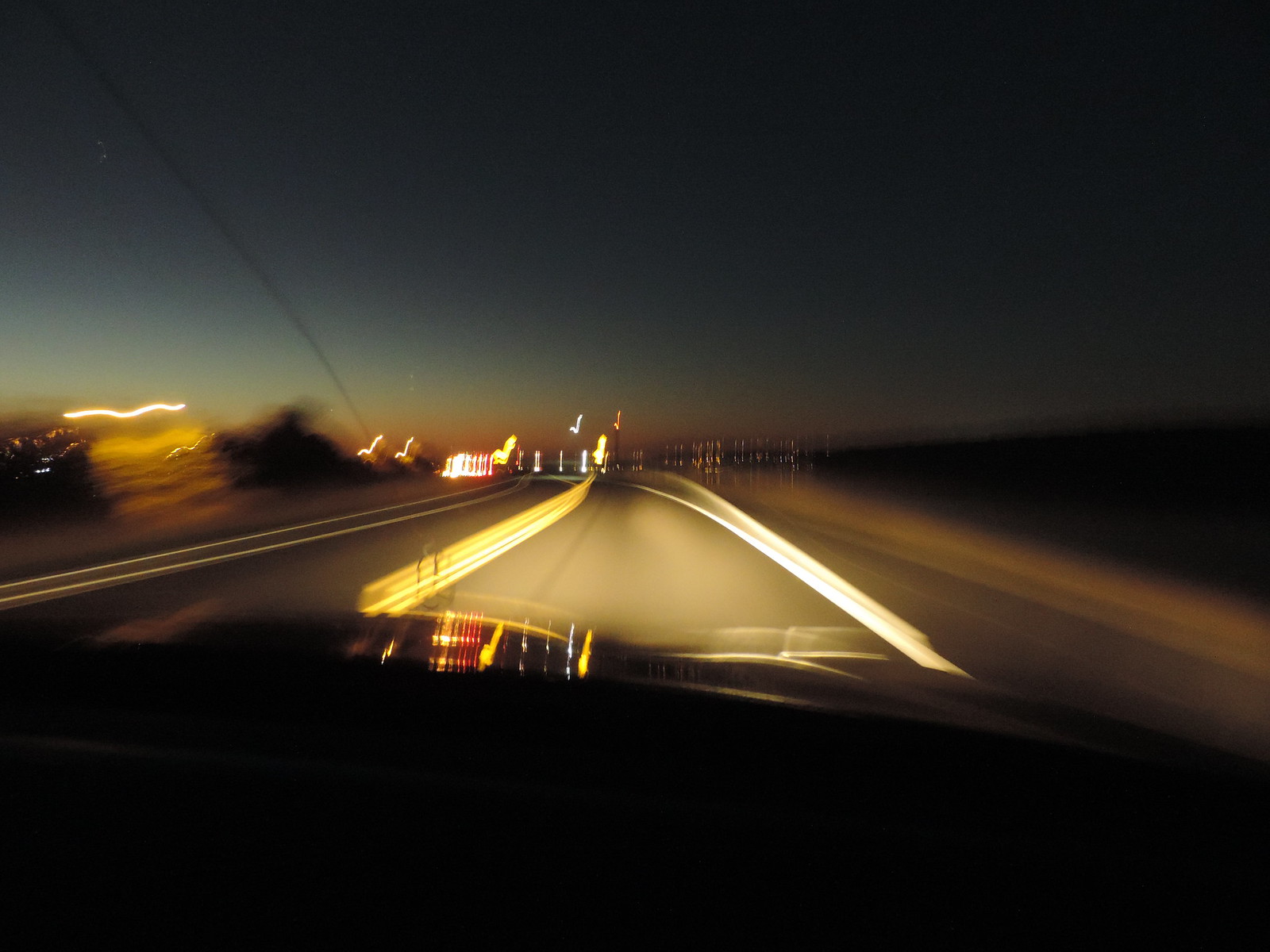This image captures a blurry nighttime scene from inside a car, likely from the passenger seat, driving down a two-lane road. The windshield and dashboard of the car are visible at the bottom of the photo, both exhibiting a significant level of blur. The photograph appears to be taken around twilight or dusk, indicated by the faint light on the horizon and the darkened sky above. The road ahead, partially illuminated by the car's headlights, shows a center line separating the lanes and a right-side boundary line, and it seems to bend to the right in the distance. Various lights from buildings or streetlights dot the horizon, and these, along with any other light sources, appear warped and streaked, likely due to an extended exposure time or camera movement. The overall effect suggests a sense of motion and a transition from day to night, possibly capturing the initial emergence of stars in the sky.